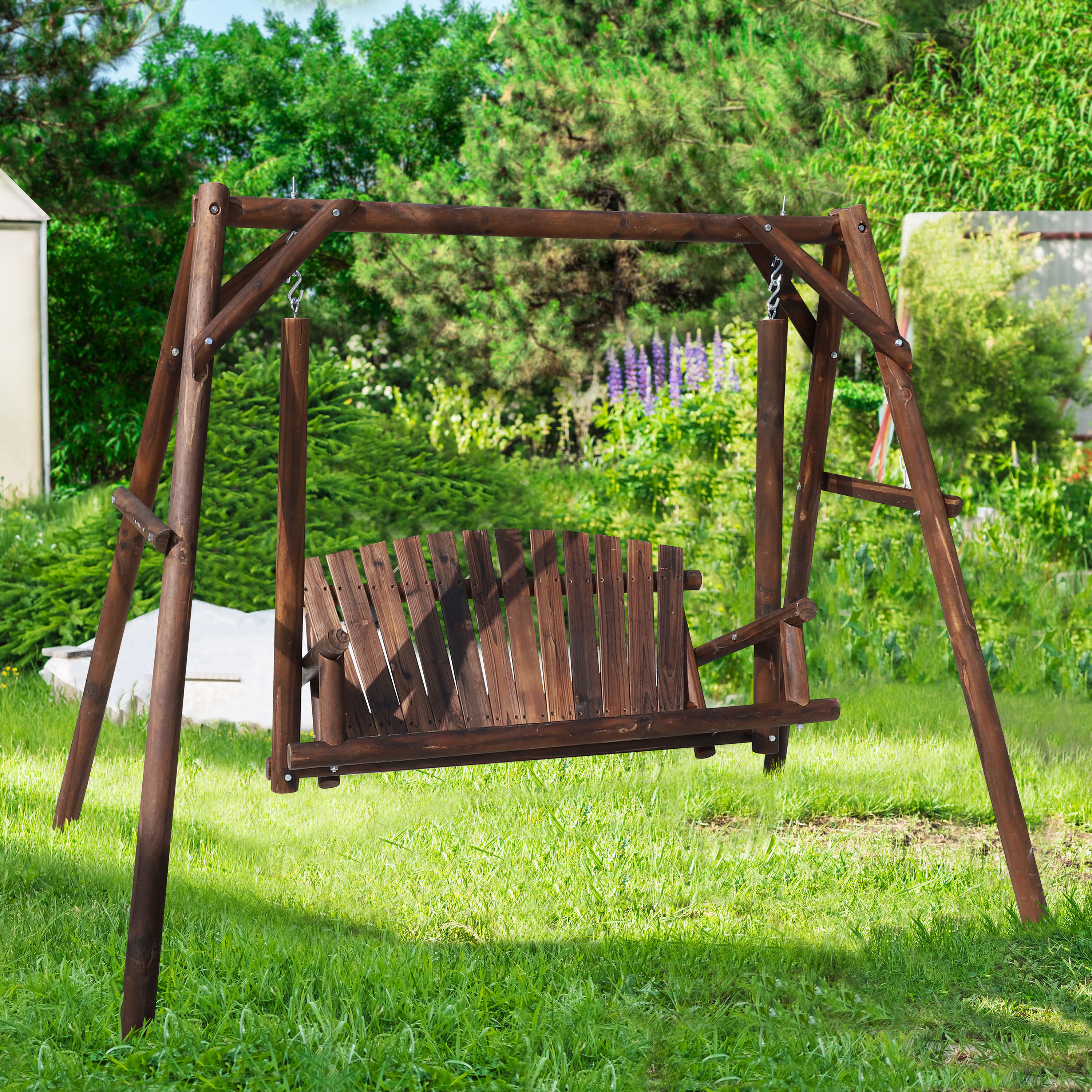This image captures a serene backyard scene featuring a dark-stained wooden swing, large enough to comfortably seat two people. The swing hangs from sturdy metal chains and sits amidst a vibrant, green lawn. Behind the swing, a mix of lush, green vegetation is visible, including various bushes, hedges, and trees, specifically pine trees. Splashes of purple from tall, vertical flowers, possibly foxtail lilies, add a striking contrast to the greenery. In the background, there's a partial view of a building, possibly a storage shed or a home, as well as another roof structure, which might be a barn or additional storage space. The sky, peeking through the foliage, is a mix of light blue and gray hues, suggesting a tranquil day. The setting exudes peace and natural beauty, perfect for relaxation.